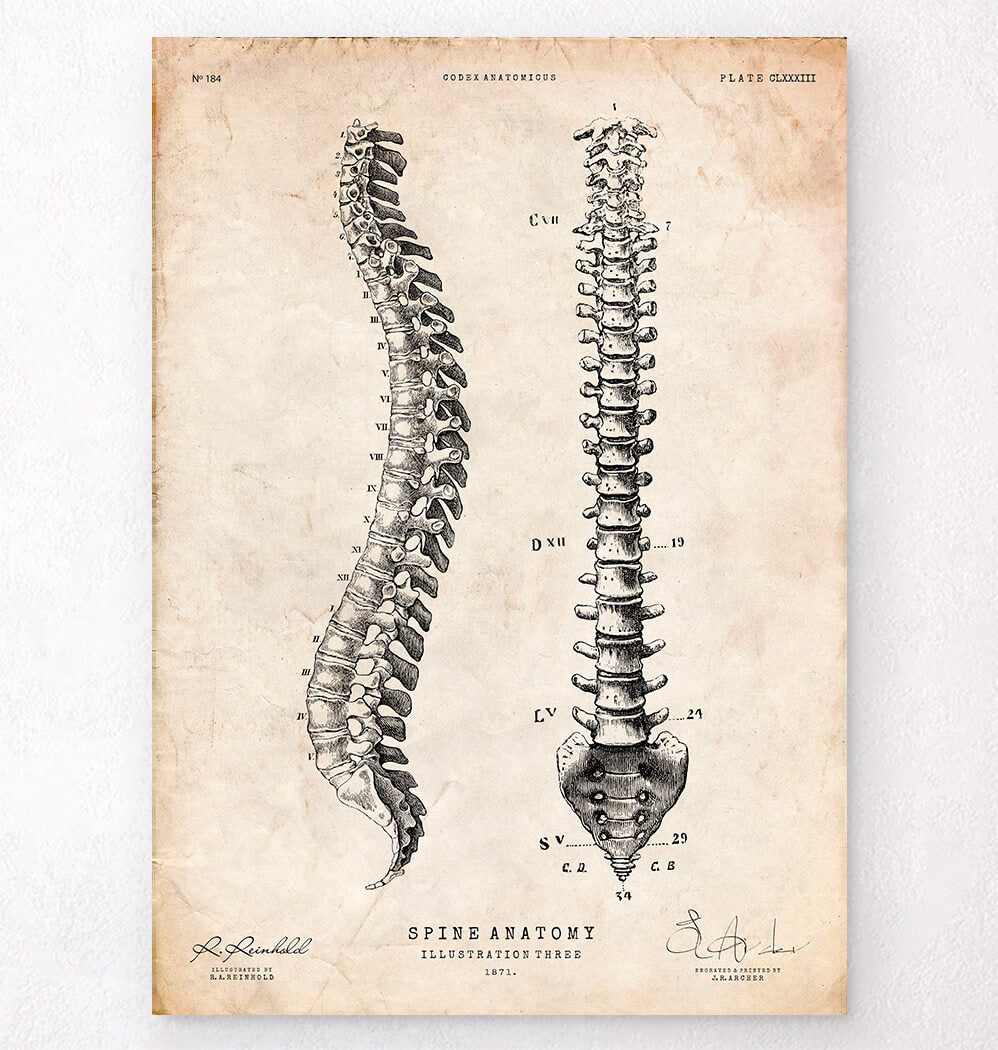The image depicts an intricately detailed anatomical illustration of a spine from an 18th-century perspective, presented on a light brown, slightly aged paper with white highlights. In the center, the paper features two views of the spine side by side; on the left is a side view of a spine, elegantly curved in an S-shape, labeled numerically from 1 to 7 and I to XX, with a pointed, slightly left-curved tail. On the right is a front view of a spine, straight and composed of small, cube-shaped bones with slight protrusions at the edges, culminating in a triangular-shaped base. At the bottom center, the text "Spine Anatomy" is clearly visible, accompanied by additional text indicating "Illustration 3, 1871." The top part of the image presents the title "Codex Anatomicus" in black ink, while "Plate CLXXXIII" and number "184" are positioned at the top right and left corners respectively. The paper, containing signatures and further annotations on either side, appears to be set against a grey background, bringing out its historical aura with shades of palish yellow, black, grey, and white.